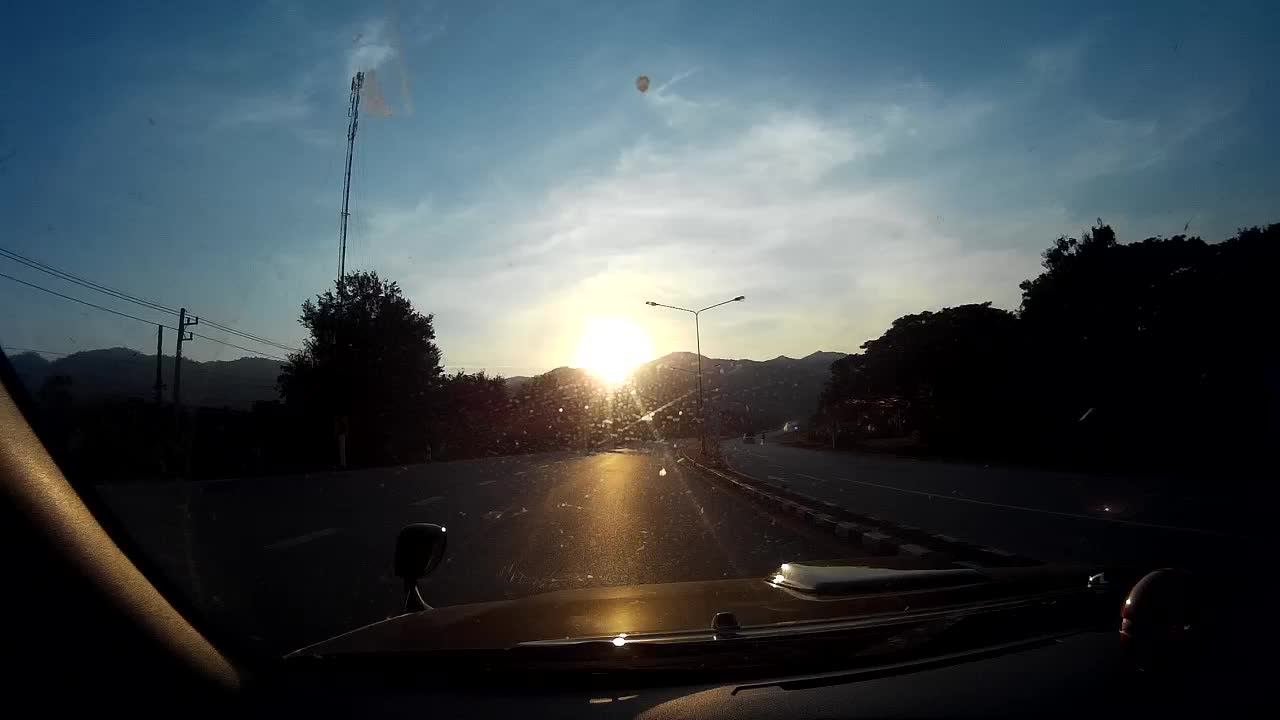This photograph, taken from inside a car looking through its windshield, captures a vivid sunset scene. The car appears to be driving down a divided road with a cinder block median. The setting sun blazes brightly on the horizon between two distant mountains, casting a harsh, blinding light that washes out many of the image's colors. Tall street lamps line both sides of the road, their lights poised to shine down. Power lines and a large antenna can be seen on the left side, stretching above the silhouetted treetops. The hood of the car, colored in a reddish-orange, features mounted lights and a spoiler, adding detail to the foreground. In the bluish sky, streaked with wispy clouds, an unexpected hot air balloon floats near the top of the image, adding an element of intrigue to the otherwise sunset-dominated scene.